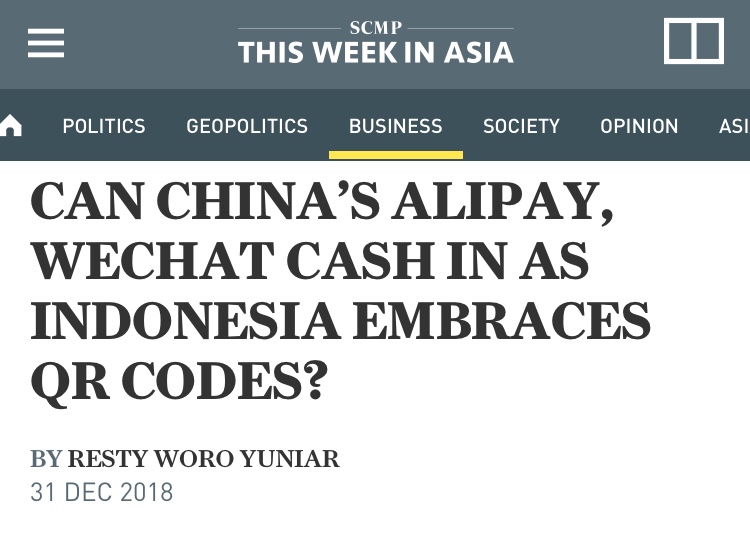Detailed Caption:

This image features a promotional graphic with a white background. Prominently displayed at the top is the logo for "SCMP This Week in Asia." Below the logo, there are several category headers including "Politics," "Geopolitics," "Business," "Society," and "Opinion," with "Business" notably underlined in yellow. Alongside these headers, a small hamburger menu icon and a square icon are visible.

The headline in bold black text reads: "Can China's Alipay and WeChat Cash In as Indonesia Embraces QR Codes?" Below this headline, the author's attribution is written in gray text: "by Rusty Worouyar." Just beneath the author's name, the date "31 December 2018" is also displayed in gray.